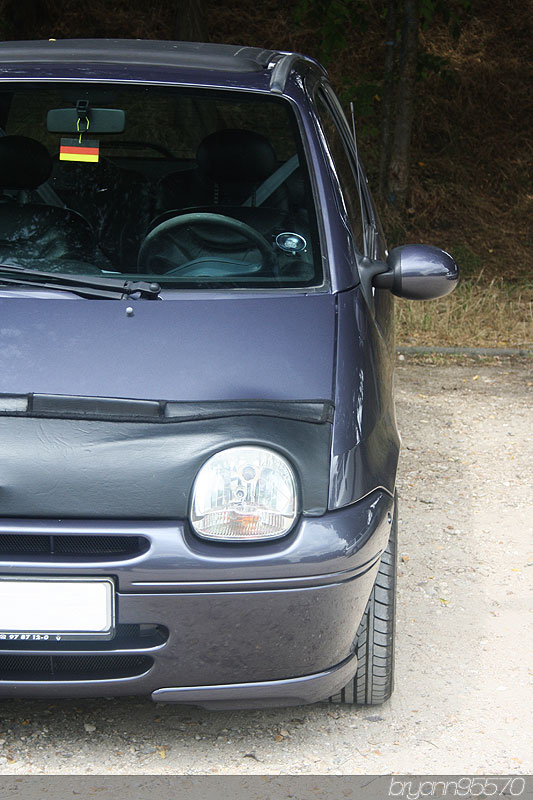A photograph captures the front half of a small, dark gray-blue two-door compact car, parked in a gravelly area within a park-like setting. The car's sleek and clean appearance is accentuated by a leather or material covering along the front of the hood and around the headlight. Prominently visible is the driver's side door and a distinct headlight, as well as a plain white rectangle where the license plate would typically be. Hanging from the rear view mirror is a rectangular flag with horizontal black, red, and yellow stripes, likely representing Germany. The interior, which appears dark, includes a dark-colored steering wheel and seating. In the background, trees and dry grasses rise on an embankment, adding a natural touch to the scene. The lower part of the image is marked with the text "BRYANN95570."